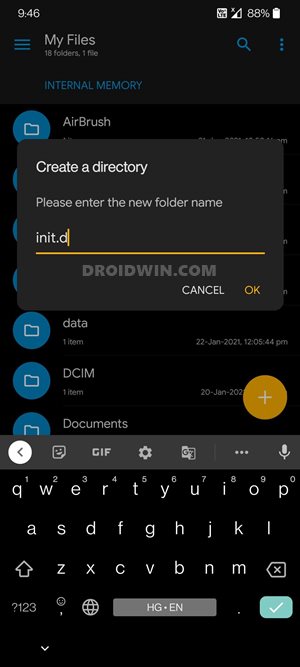"Screenshot from a smartphone with a black background, showing the time as 9:46 in the upper left corner. To the right, there are several icons, including a square, signal strength, '88%' battery percentage, and a battery icon.

Below the time, there are three horizontal blue lines, indicating a menu. The title 'My Files' displays with '18 folders' and '1 file' underneath. On the far right, a magnifying glass search icon is followed by three vertical dots for more options.

The screen displays sections, starting with a blue circle featuring a white file icon labeled 'airbrush', followed by several similar icons partially obscured by a light black square. The overlay square contains the text, 'Create a directory. Please enter the new folder name', with 'init.d' being typed in. Below this prompt, an orange line reads 'droidwin.com'.

At the bottom right, there are 'Cancel' and 'OK' buttons. Below this, visible folders include one labeled 'Data' with a single item, dated 22nd January 2021 at 12:05:44 PM, followed by 'DCIM', with its date partially cut off by an orange circle with a white plus sign. The last visible folder is 'Documents'.

A gray line separates the folders from various icons including a left arrow, smiley face, GIF icon, gear, Google 'G', three horizontal dots, and a magnifying glass. Below these icons, the QWERTY keyboard layout is visible, showing keys 'QWERTYUIOP' with secondary number labels '1-0', followed by 'ASDFGHJKL', and the bottom row starting with an upward arrow, 'ZXCVBNM', and a delete key. The last row groups keys including '?123', emoji, globe, space bar labeled 'HG star EN', period, and an aqua blue button with a white check mark, ending with a single down arrow button."